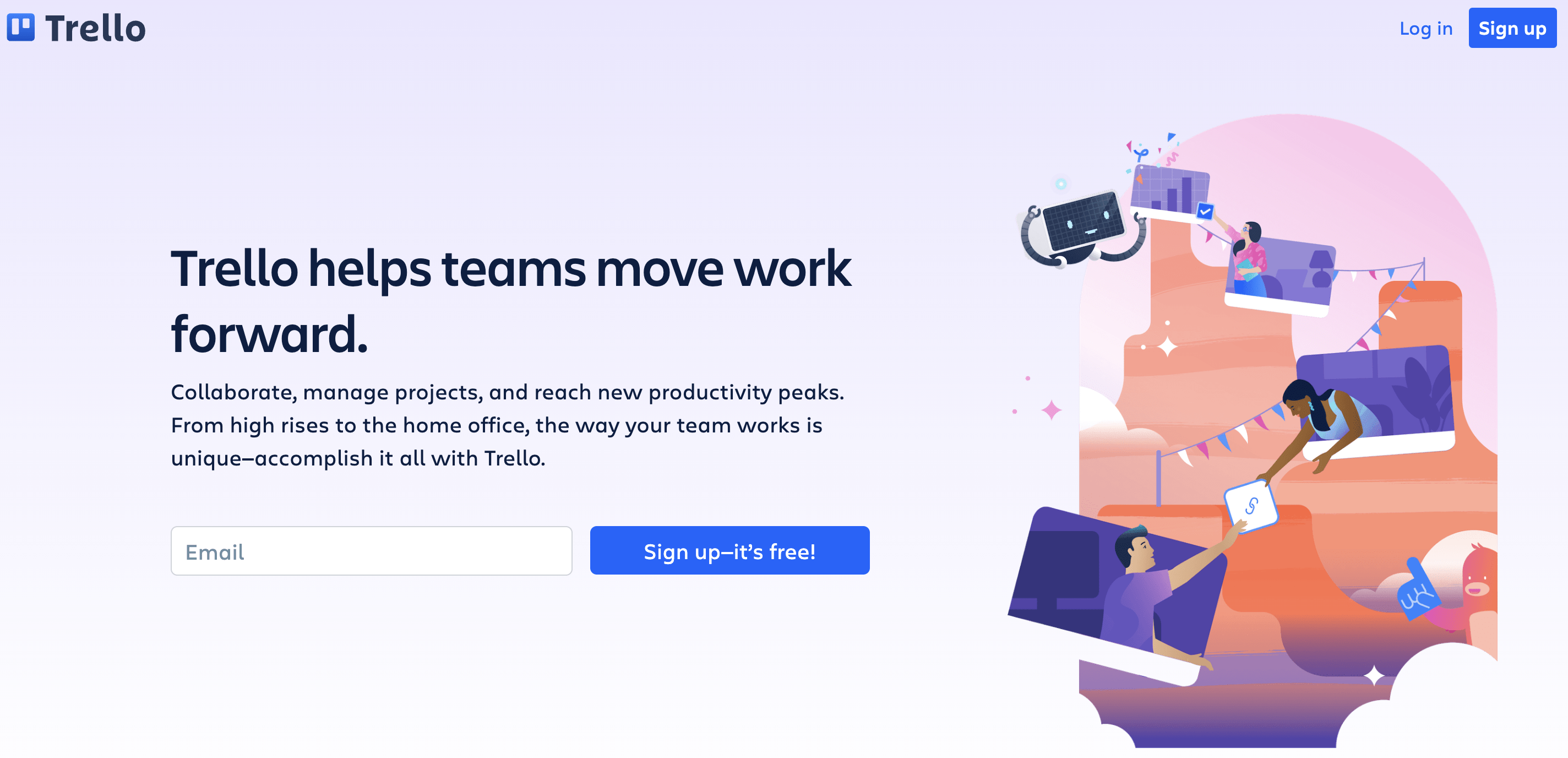**Detailed Caption:**

The image is from the website Trello, prominently indicated by the text "Trello" in the upper left-hand corner. Adjacent to the text is a blue square containing the company’s logo, which features two vertical white lines, the left line being longer than the right. The entire image is rectangular, approximately twice as wide as it is tall, set against a pale lavender background.

On the left side of the image, just above the center, bold black text reads, "Trello helps teams move work forward." The only capital letter is the 'T' in "Trello." Beneath this line, in smaller black text, it further explains, "Collaborate, manage projects, and reach new productivity peaks. From high rises to the home office, the way your team works is unique - accomplish it all with Trello."

Below the text description is a white rectangle intended for users to input their email address, identified by the word "Email." To its right lies a blue rectangle button with white text that reads, "Sign up - It's free!" Additionally, in the upper right-hand corner, there’s a blue rectangle with white text saying "Sign up," and to its left, "Log in" is written in blue against the lavender background.

The right-hand one third of the image is illustrated. It features a backdrop of a pink arch and various purple areas resembling computer screens. In the bottommost screen, a man in a purple t-shirt is reaching up and handing a woman in a blue dress, who is in a screen above him, a white square with a blue outline. Above them, another woman in a pink shirt hands an item upward within other screen-like areas. A small black figure resembling a robot, with a rectangular head, blue eyes, and a blue smiling mouth, reaches its arms upward on the left. The background behind these screen-like shapes transitions through muted shades of orange and culminates in a blend of purple and orange at the bottom.